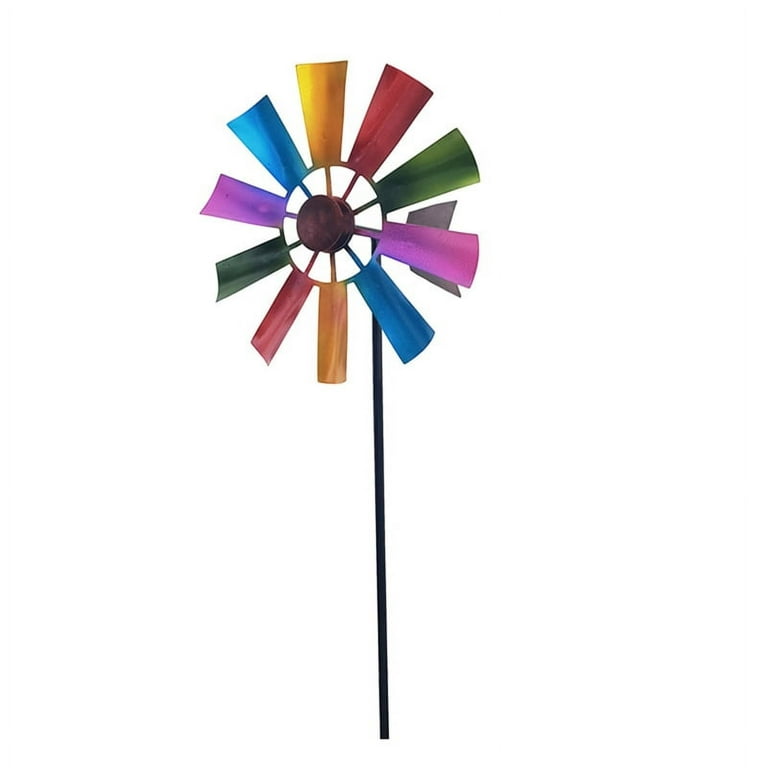The image depicts a colorful garden windmill ornament against a plain white background. The windmill features a thin black rod that stands vertically and then bends at a 90-degree angle to support the circular fan mechanism. The fan itself comprises an inner circle, or hub, with ten multicolored blades radiating outward, each alternating in shades of green, purple, blue, orange, yellow, and red. These blades have a metallic appearance, resembling anodized titanium, giving off a reflective sheen. At the center of the fan is a brownish-black disc that secures the blades in place. Surrounding the blades is an outer circular frame to which they are connected by spoke-like bars, each colored to match the respective blade it supports. This windmill, designed to be placed in the ground, perhaps in a flower pot, presents a vibrant and decorative garden feature.